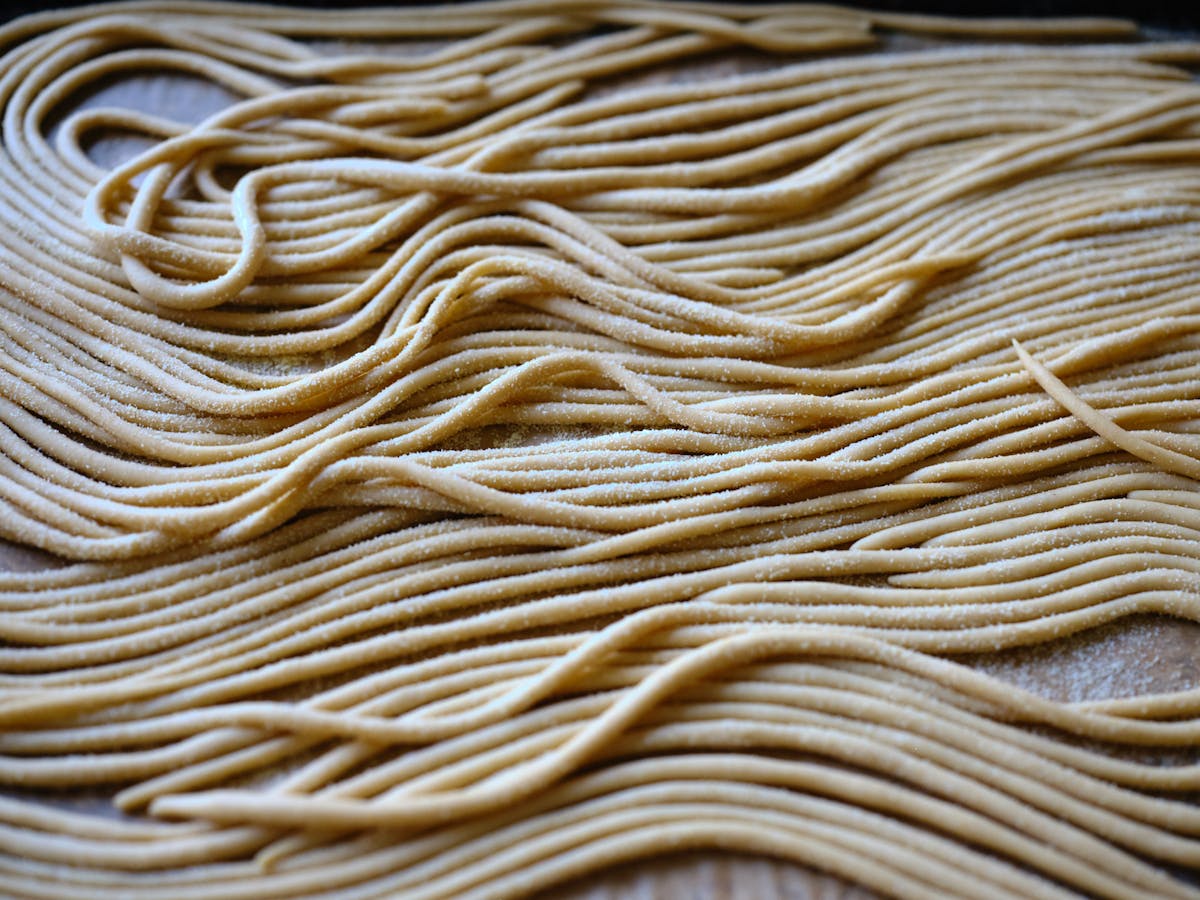This image showcases a close-up view of rows of thin, string-like, light tan-colored homemade pasta noodles, resembling spaghetti, spread across a wooden surface. The surface and noodles are lightly dusted with a granular substance, likely flour but potentially sugar or salt, contributing to a lightly coated appearance. The noodles are uniformly arranged, long, and slender, typical of spaghetti width and color, suggesting they might be prepared for an upcoming dish.